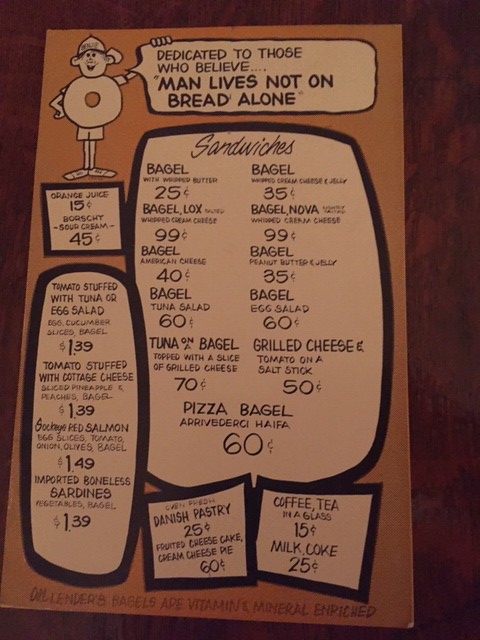This image features a vintage-style menu with a light brown background and dark brown text. The text is set against a light tan backdrop, creating a visually distinct and readable layout. 

At the top left corner, there is a whimsical cartoon character: a man wearing a cap, characterized by a circular torso resembling a cheerio. The character's right hand rests on his hip, while his left hand holds out a speech bubble saying, "Dedicated to those who believe man lives not on bread alone."

Beneath the cartoon, in a creatively designed, organic yet rectangular box is the word "Sandwiches" written in a cursive font. Below that, listed in a straightforward Arial font are various types of bagels including "Bagel Lox," "Bagel Nova," and numerous other bagel variations.

To the left, under the cartoon character's feet, is a small box with the text "Orange Juice and Sour Cream." Directly below this is a longer rectangular box listing appetizing options such as "Tomatoes Stuffed with Tuna or Egg Salad," "Tomatoes Stuffed with Cottage Cheese," "Red Salmon," and "Imported Boneless Sardines."

Towards the bottom right of the menu are two adjacent squares. One square highlights "Danish Pastry, Cheesecake, Cream Cheese Pie," while the other square lists beverages like "Coffee, Tea, Milk, and Coke." 

The prices on the menu are quite nostalgic, ranging from 15 cents for Coffee and Tea to $1.49 for Red Salmon.